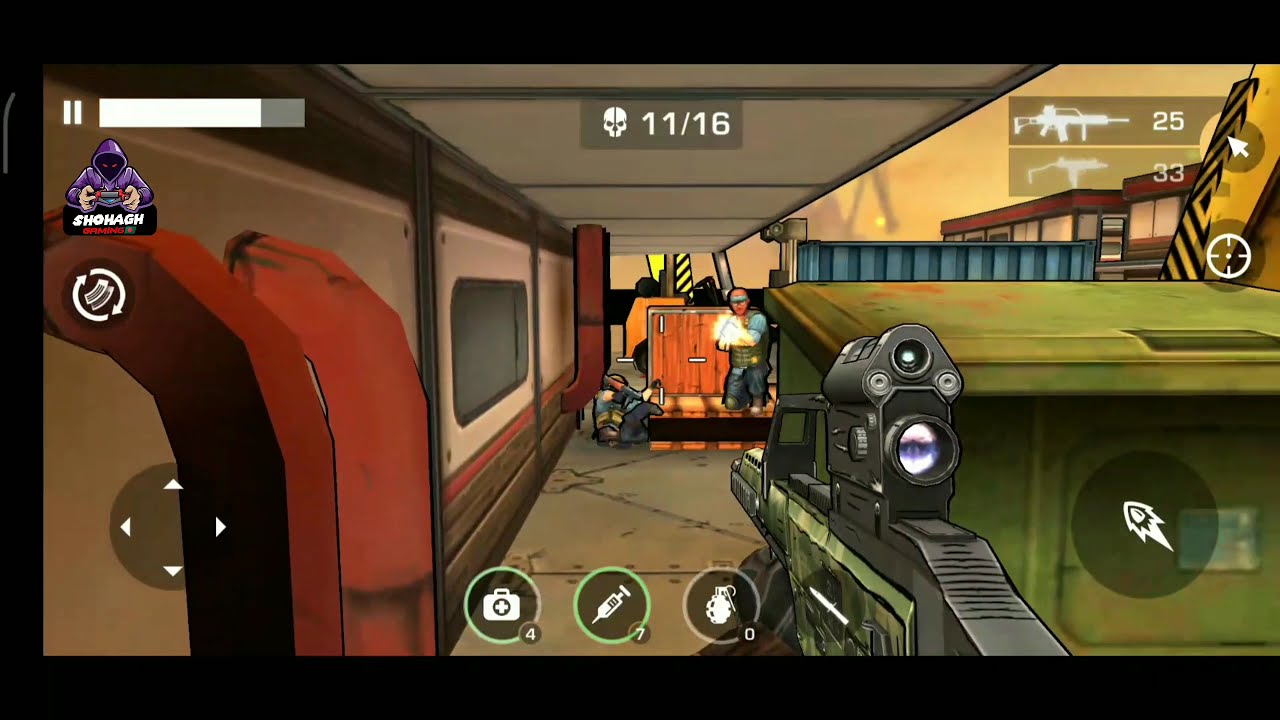This is a highly detailed screenshot from a first-person shooter mobile video game, presented in a horizontal rectangular format. The foreground prominently features a tank or armored military vehicle on the right side. On the left, there's a distinctive brown and orange archway leading to another room. Beyond this, a tan wall with a screen is visible. In the background, a man wearing a white shirt and jeans is standing on what appears to be a forklift. The game interface is rich with details: a white progress bar and status icon are at the top left, along with a pause button. The top right displays two weapon icons, one resembling a rifle with an ammo count of 25, and another with a count of 33. A skull icon in the middle top of the screen shows a kill count of 11 out of 16. The lower left corner features a transparent overlay of a game controller or directional pad. At the bottom center, three white-outlined circles denote a first aid kit, a hypodermic needle, and a grenade. A subtle, illustrative aesthetic with small black borders around in-game elements gives the screenshot a unique, almost hand-drawn appearance.